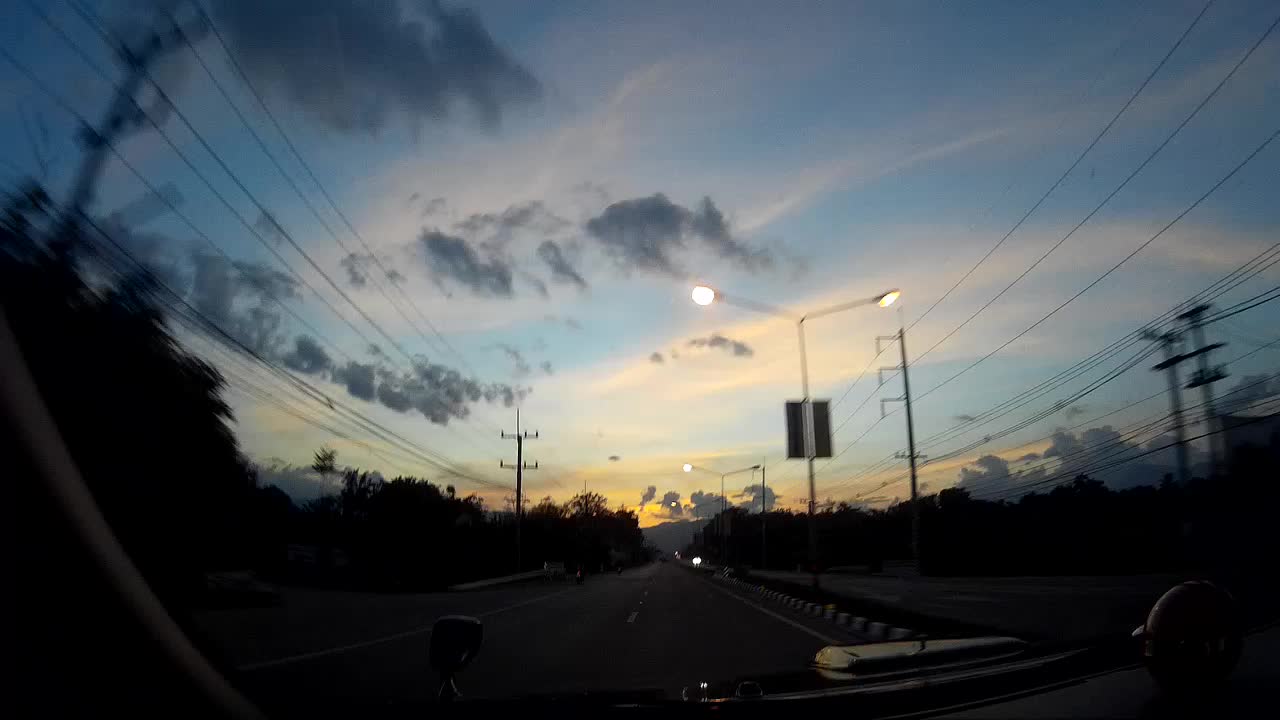This image captures a mesmerizing sunset with a unique, slightly warped perspective, likely due to a fisheye lens. The sky, predominantly a soft, lighter blue, is adorned with a mix of wispy white clouds and more ominous, dark clouds. Silhouetted against this ethereal backdrop are the outlines of trees and power lines, framing the scene. The lower half of the photograph is enveloped in darkness, rendering details of the street and surroundings indiscernible. However, the horizon is illuminated by the golden glow of the setting sun, peeking through the darker clouds at the center of the image. The vantage point suggests the picture might have been taken from a motorcycle, adding to the spontaneity and dynamic feel of the scene.